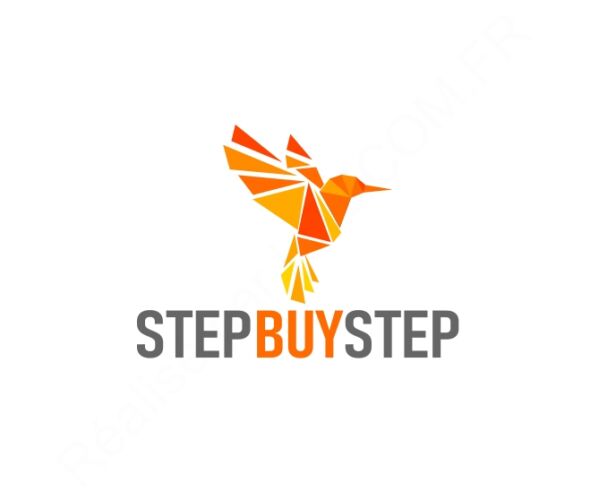In the center of this image, set against a completely white background, is a striking and colorful logo in the shape of an abstract bird, facing right with its wings extended upward to the left. This bird is composed entirely of various triangles, creating an intricate mosaic. The top part of the bird's wings features a gradient of red, orange, lighter orange, brighter orange, and yellow, while the body incorporates shades of yellow and brown. The beak stands out in orange. Beneath this artistic depiction, the phrase "STEP BY STEP" is written in all capital letters, with "STEP" in grey and "BY" in orange. This minimalistic yet vibrant logo, likely designed for a company, effectively uses geometric shapes and a limited color palette to create a memorable visual impact.